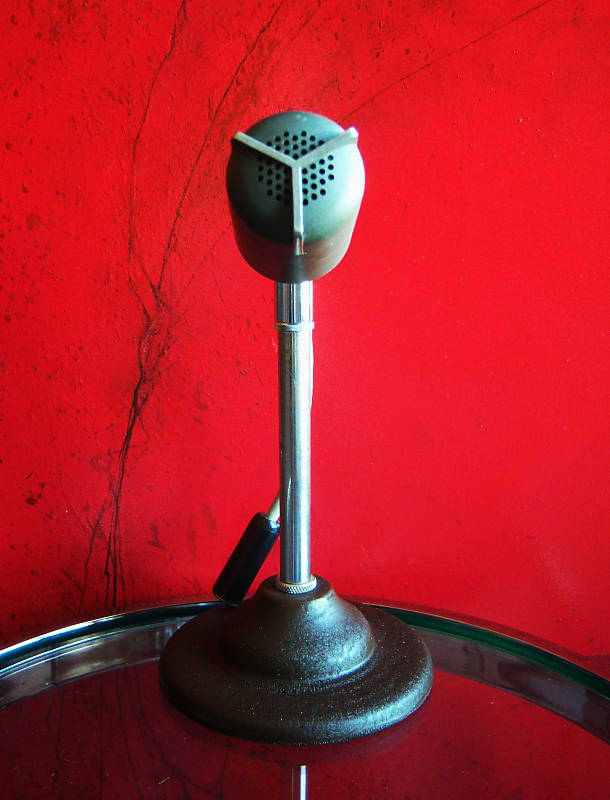This photograph features a vintage microphone with design elements reminiscent of those used by singers from the 1920s through the 1950s. The microphone has a distinctive raised Y shape at the center of its gray front, which is perforated with numerous holes. It is mounted on a thin cylindrical metal stand, which is affixed to a black, almost conical base. This structure stands on a glass table, partially framed by a metal outer ring. The background is striking and artistic, consisting of a deep red wall adorned with black lines, streaks, and splotches, reminiscent of brush strokes or scratches, adding an element of visual intrigue to the scene. A wire extends from the microphone's rear, covered by several black cylindrical elements. The overall color palette of the microphone includes shades of gray, silver, black, and hints of an aged copper-like greenish-blue, contrasting sharply against the vivid red backdrop.